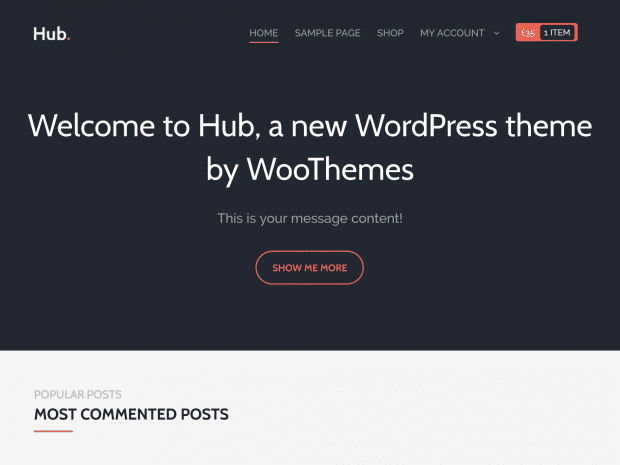This is an image from my website titled "Hub". On the top left, there's a navigation menu featuring buttons for "Home", "Sample Page", "Shop", "My Account", and "Item". Just below this menu, the heading "Welcome to Hub" is prominently displayed in white font, accompanied by a subheading that announces "A new WordPress theme by WooThemes". Beneath this, the text "This is your message content!" is also in white. Another focal point on the page is a noticeable "SHOW ME MORE" button – the text is bold, in all capital letters, and in red, encapsulated within a circle. Further down the page, the section titled "POPULAR POSTS" catches the eye, followed by another section labeled "MOST COMMENTED POST", both in all capital letters. A striking red line divides these sections, adding a clear visual separator.